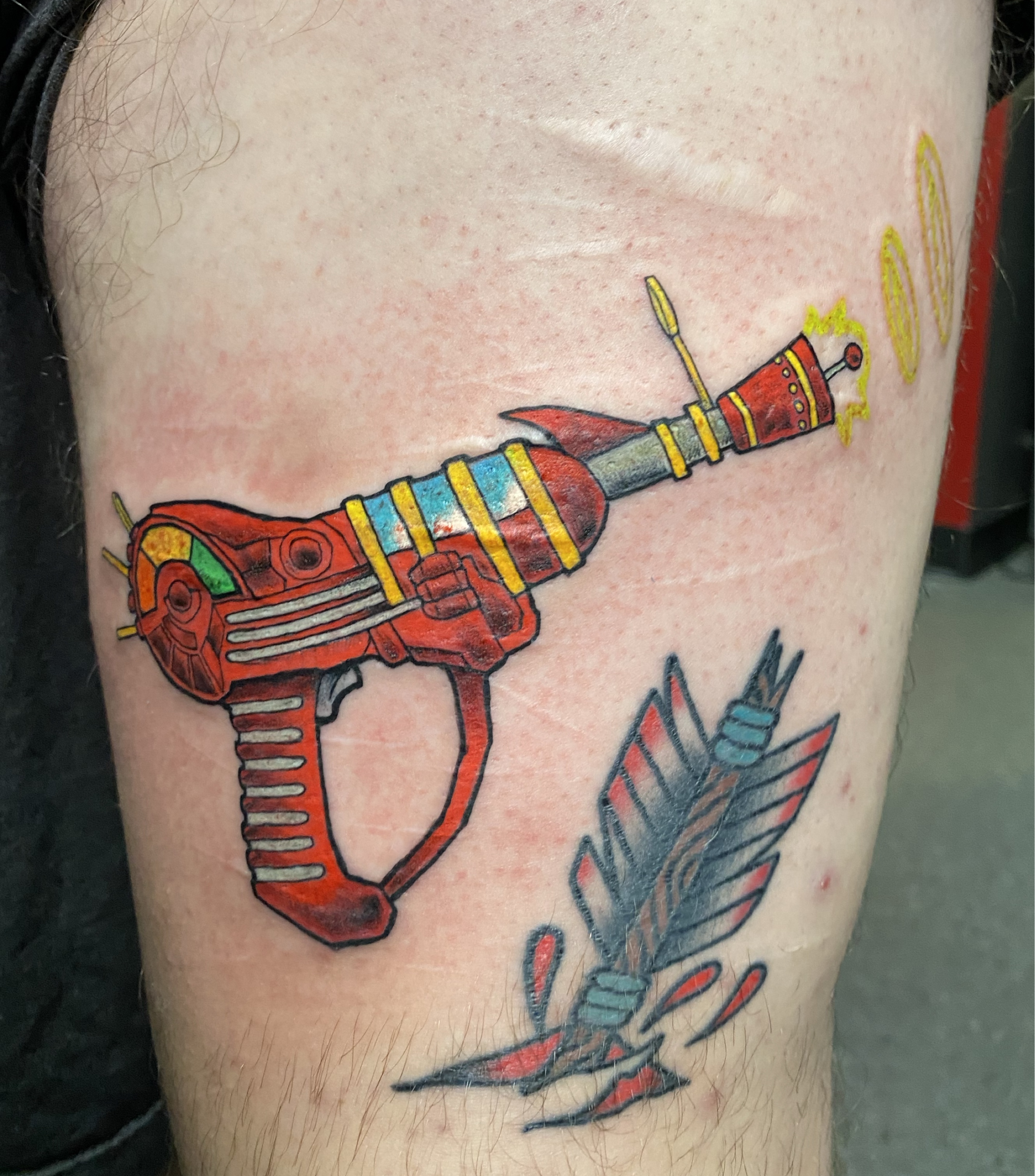This color photograph features a close-up of a Caucasian man's upper leg, revealing two intricate and colorful tattoos on shaved skin. The upper tattoo, situated just below the knee, depicts an animated, toy-like laser gun. This fantastical weapon boasts a vibrant palette, with a primarily orange body adorned with gold bands and gray stripes on the handle. The barrel transitions to a red tip, emitting yellow rays, and features blue segments, adding a futuristic flair. Below this, another tattoo portrays an arrow seemingly piercing the skin, complete with blood drops to enhance the illusion. The arrow, designed with brown and blue hues, showcases red-tipped feathers tied with blue rope, giving it a dynamic, almost lifelike quality.